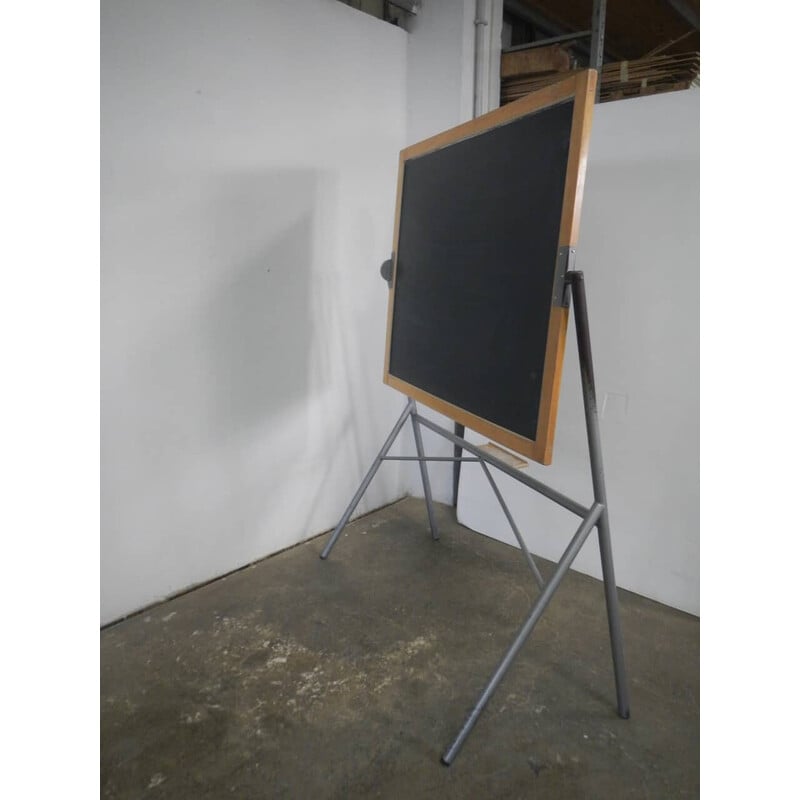In the corner of a sparse, warehouse-like room with white walls and a gray, slightly dirty concrete floor, stands an empty black chalkboard with a tan wooden frame. The chalkboard is supported by metal brackets and poles that form an A-shaped base, with one leg angled and the other vertical. Positioned against a white wall, there is an opening or window above the chalkboard showing wooden slats outside, providing a glimpse of some brown hues amidst the predominantly monochromatic setting. In the upper right corner, some cardboard and a metal rack or easel can be seen, adding to the utilitarian feel of the space.